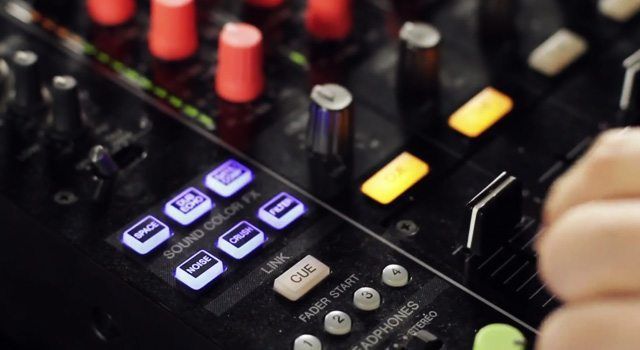The photograph captures a detailed, close-up view of a musical soundboard, likely used for DJ performances or recording sessions. The image is a rectangular indoor shot, approximately four inches wide and three inches high, with a black plastic panel hosting an array of controls. Predominantly black, the soundboard features numerous knobs and buttons with various functions.

In the lower right-hand corner of the image, a person's hand, showing just three fingers, manipulates a volume slider. The hand appears to belong to a person of Caucasian descent.

Starting from the top left of the soundboard, there are two thin, tall cylindrical knobs with silver tops. Below these knobs, a switch is flipped to the left. Continuing downward, the panel contains six buttons labeled "Sound Color FX." The first row of three includes an illuminated white button labeled "Space," while the identities of the remaining two buttons are obscured by the photograph's focus. The second row features buttons labeled "Noise," "Crush," and "Filter," though “Crush” and “Filter” are somewhat out of focus. Below these rows is a single illuminated white button labeled "Cue," and under it, the words "Fader Start" with four non-illuminated buttons labeled 1 to 4.

On the upper right section of the soundboard, the panel contains a series of five large red turn knobs. Below them are two silver knobs with their indicators pointing upwards. Adjacent to these are four buttons—two illuminated yellow and two white, which are not illuminated.

Towards the bottom of the image, just above a truncated view where the letters “H” and “E” of the word "Headphones" are cut off, another slider is present with the label "Stereo."

Overall, the photograph provides a detailed, albeit slightly blurred, look at a sophisticated electronic soundboard designed for intricate sound management, accentuated by various knobs, buttons, and sliders intended for creating dynamic audio effects.